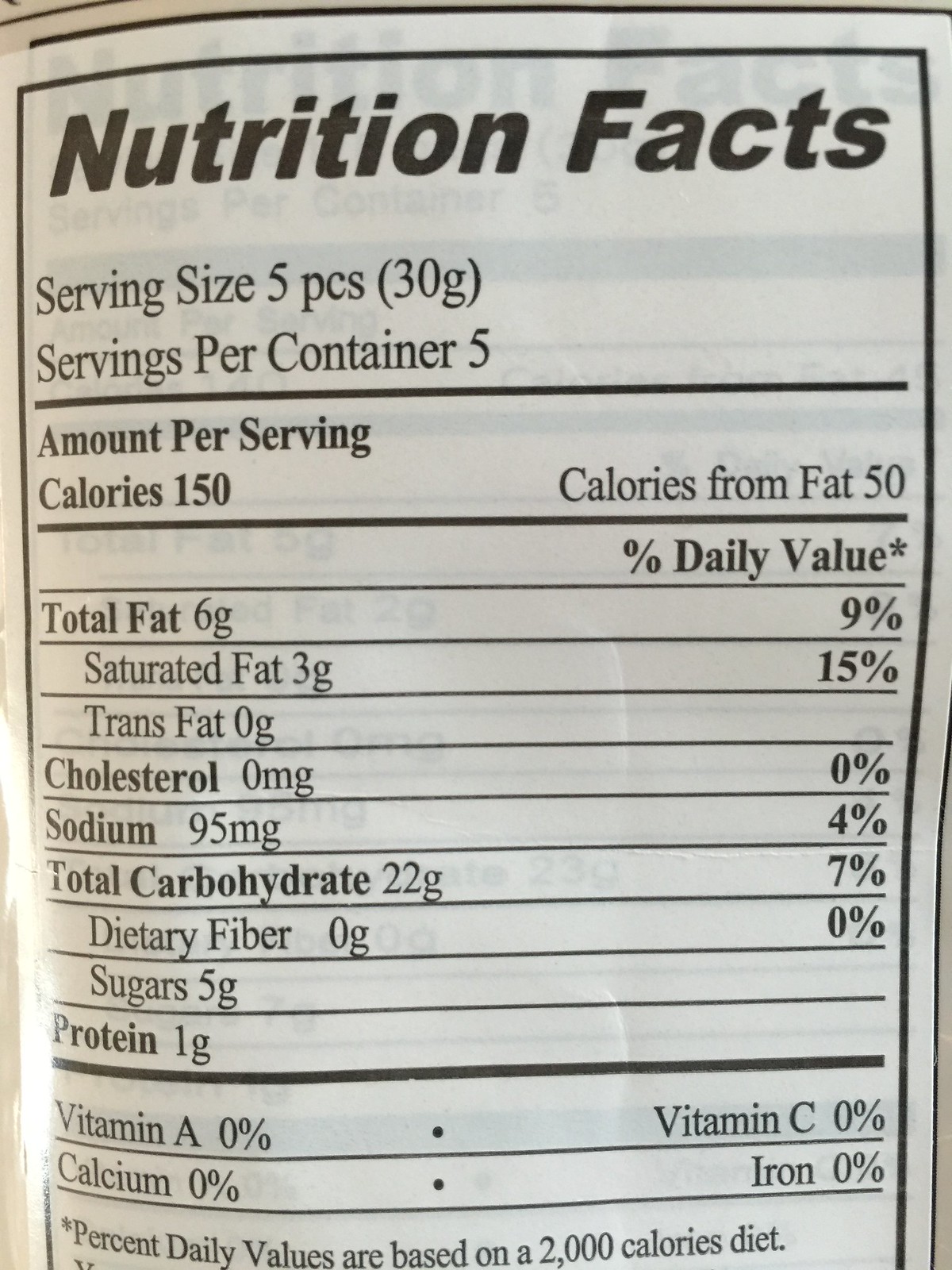This image displays the nutrition facts for a product, written in black lettering. The serving size is specified as five pieces, weighing 30 grams, and there are five servings per container. Each serving provides 150 calories, with 50 of those calories coming from fat.

The total fat content is 6 grams, representing 9% of the daily value. Saturated fat amounts to 3 grams, which is 15% of the daily value, while trans fat is negligible at 0 grams. The product contains no cholesterol. The sodium content is 95 milligrams per serving, making up 4% of the daily value. 

In terms of carbohydrates, each serving contains 22 grams, equivalent to 7% of the daily value, with 0 grams of dietary fiber and 5 grams of sugar. The product does not provide any significant amounts of Vitamin A, Calcium, Vitamin C, or Iron.